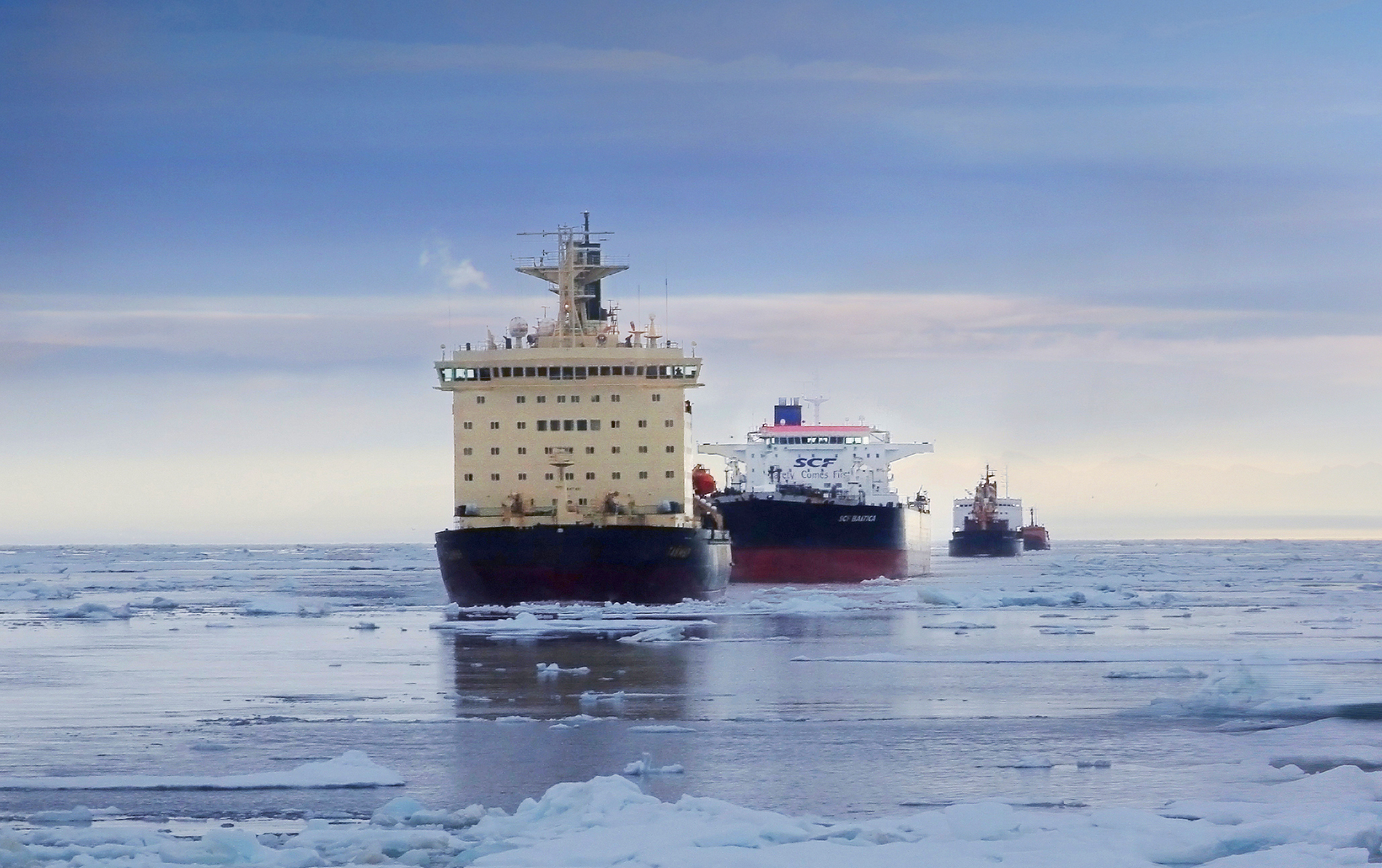This photograph captures a serene yet dramatic scene in what appears to be the Bering Sea, where several boats navigate through ice-filled waters. The composition is divided into three distinct layers: the top third of the image showcases a vivid blue sky, transitioning to a whitish middle section with scattered clouds. The bottom third features a calm, flat ocean, punctuated by floating ice in the foreground.

Prominently, two large boats stand in the foreground. One of them, facing away from the viewer, has a black hull and a superstructure that rises straight up in a white or beige color. This boat features four rows of windows, crowned by an upper area with additional windows—resembling a cruise ship, although its proportions suggest otherwise. The second boat, slightly behind the first, has a striking red lower hull transitioning into a black section, much like the traditional colors of the Titanic. Above the black, the boat has a white upper section marked with the letters "SCF" in blue on the back.

In the distance, two more boats are visible, creating a procession through the icy waters. The third boat in line sports a black hull and a white superstructure, while the fourth and most distant boat appears predominantly black. All these vessels seem to be following a navigated path through the ice.

Overall, the image captures the stark contrast between the tranquil ocean and the formidable ice, highlighting the steadfast journey of these boats through the frozen expanse.